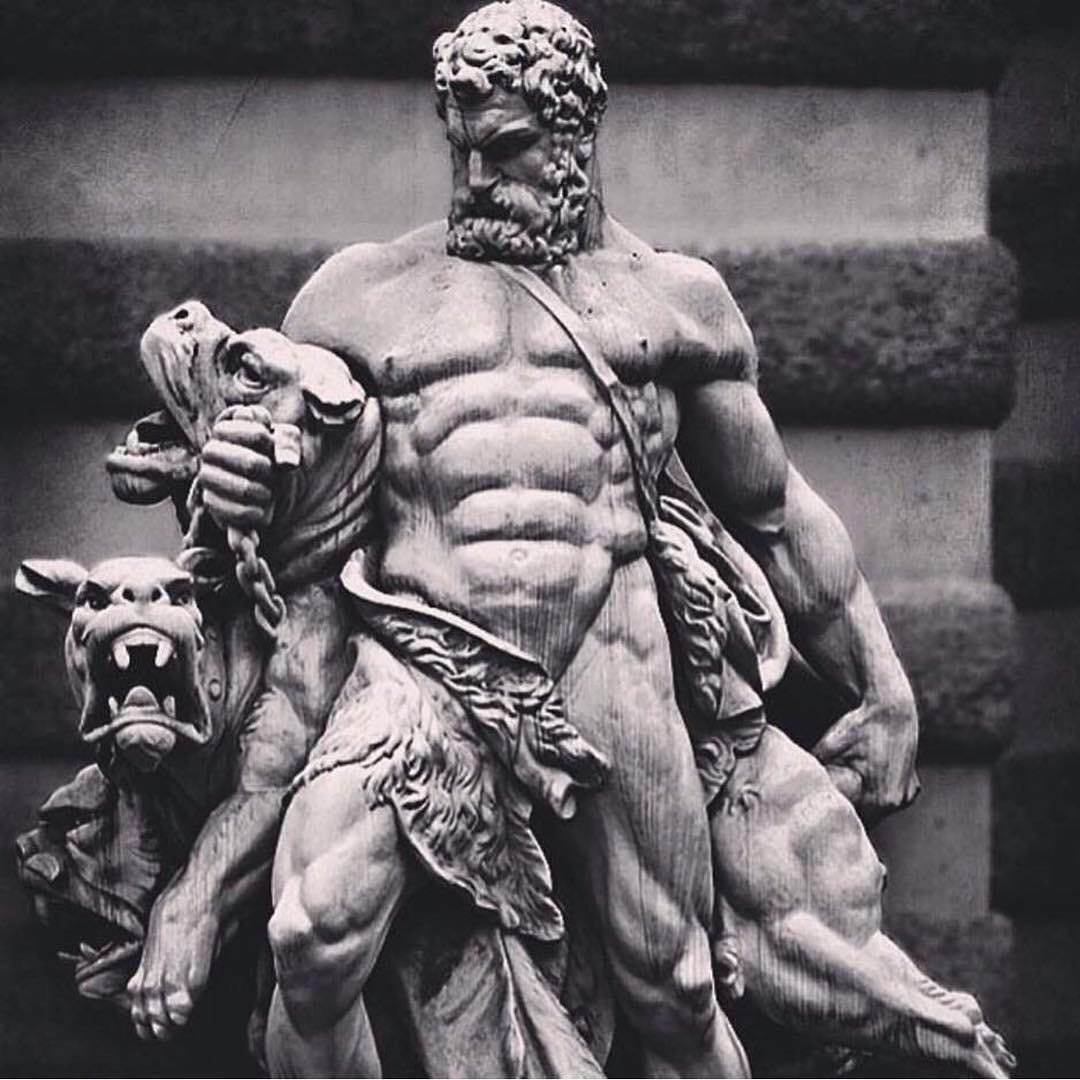The image depicts a highly detailed, close-up photograph of a stone statue set against a grayish wall with textured, dark gray stripes adding depth and form. The central figure is an extremely muscular man, possibly a mythological figure such as Zeus, with chiseled abs, a defined chest, and robust shoulders. He has a long, curly beard and hair, and a striking Roman nose, lending him a fierce warrior-like appearance. His muscles are prominently displayed, and he's scantily clad, draped in a sheet-like fabric that covers his front. The man is gazing down at his right hand, which gripping a dog by the neck in a headlock. This dog appears wild and powerful, with its mouth open and teeth bared in a snarl. There is a chain in the man's hand, possibly part of a collar or leash. Beneath this dog, another dog faces the camera with an equally fierce, growling expression, its ears visible. The rear part of the first dog can be seen on the left side of the man's body, enhancing the dynamic and intense composition of the statue.